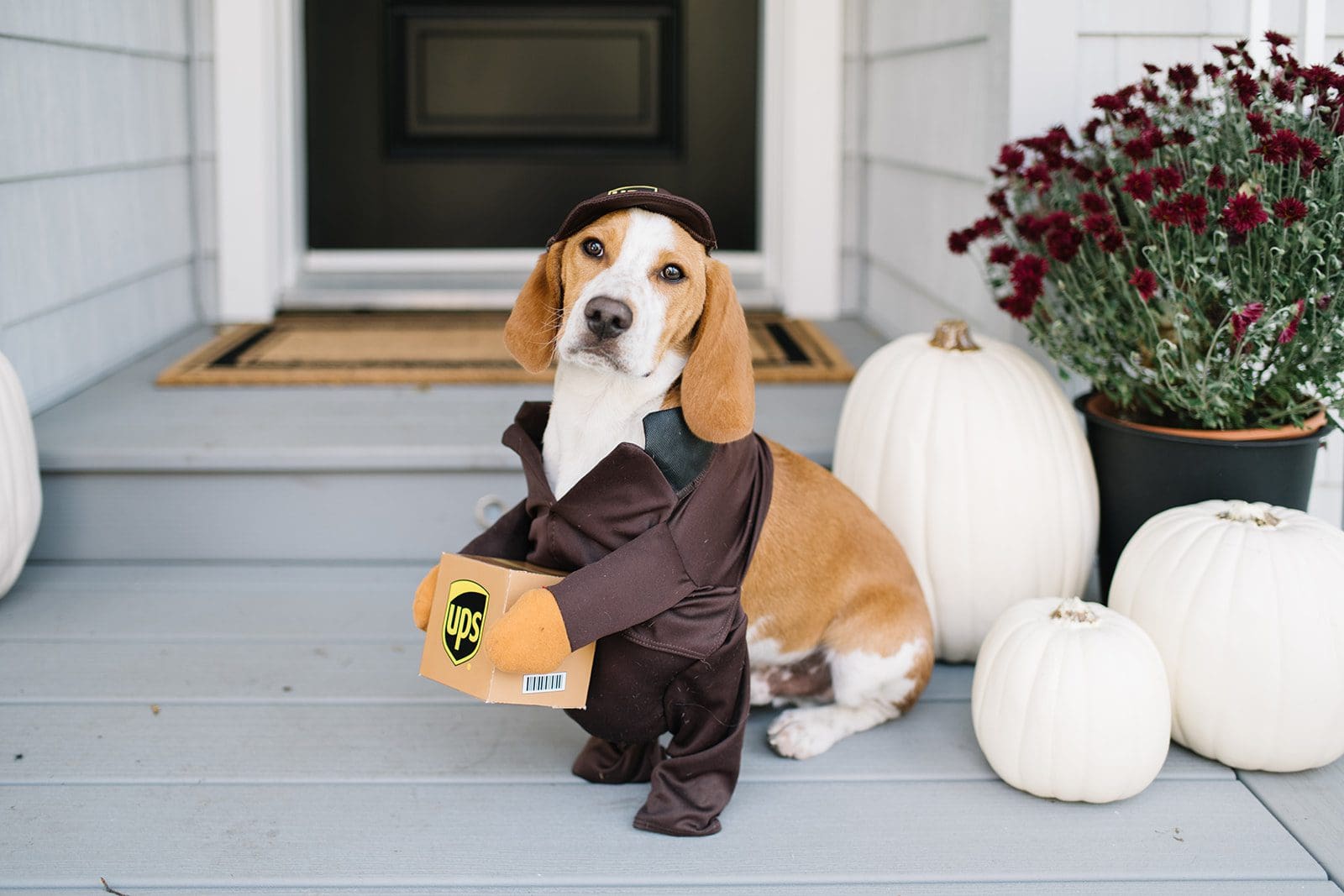In this charming landscape photograph, a beagle dressed as a UPS delivery person stands on a light gray wooden porch, directly in front of a black front door with white trim. The beagle, with his characteristic brown and white fur and floppy ears, is outfitted in an adorable brown UPS costume. The costume, fastened around the neck and chest, cleverly uses the dog’s front legs as the bottom legs of the outfit while fabric arms extend out, holding a small brown UPS box. Topping off the ensemble is a matching brown cap on the beagle's head. To the dog's right, there are three white pumpkins and a black pot filled with dark red flowers, adding to the cozy, festive atmosphere. The background reveals the gray siding of the house and a tan doormat, contributing to the overall quaint and inviting scene.